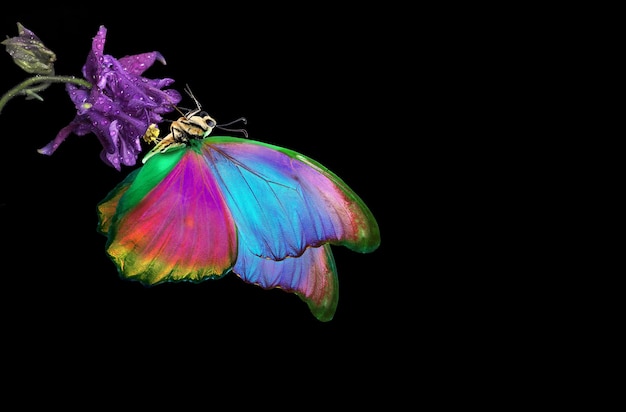This is a horizontal rectangular image featuring an artist's painting of an exquisitely colorful butterfly set against a completely black background. The butterfly's body is yellow with black accents, and it displays an array of vibrant colors on its wings, including red, pink, purple, blue, and green. The wings are notably large, especially the posterior ones, with a green outline and intricate patterns. The wings' coloration transitions, with some areas displaying bright pink fading into yellow, and others shifting from blue into purple tones.

In the upper left corner, a purple flower with numerous petals and speckled patterns hangs down, poised to interact with the butterfly. The flower is attached to a stem that is either green or brown, with a wilted leaf extending from it. The butterfly seems to be in mid-flight, moving towards the flower as if preparing to land. The delicate details of the butterfly’s antenna are subtly visible, enhancing the image's overall vividness and intricacy. This coherent composition captures a moment of delicate interaction between the butterfly and the flower, set against a stark, black background that highlights their vivid colors.